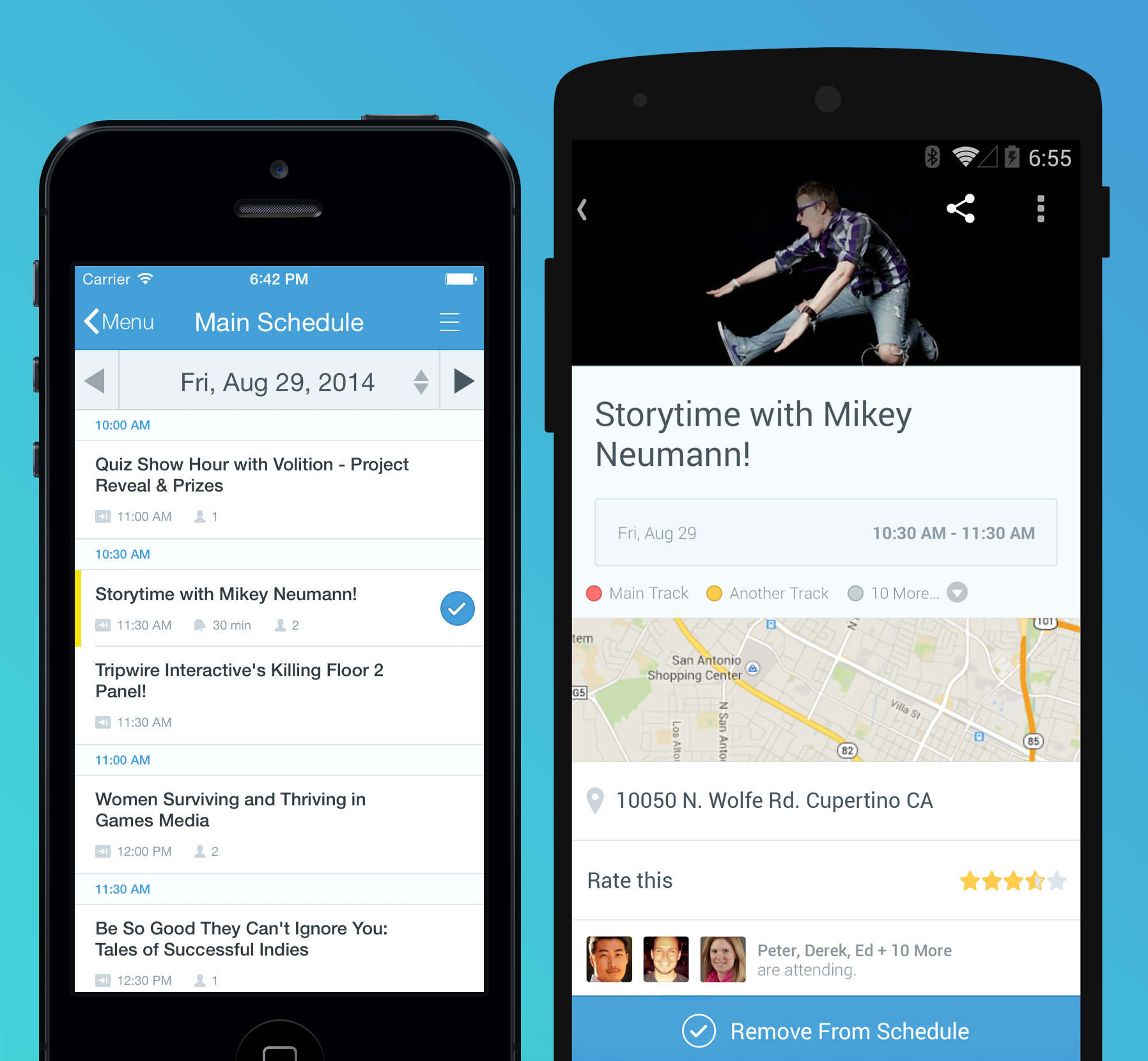The image displays two cell phones against a light blue background. On the left, there is a smaller Apple iPhone. The iPhone features a power button on the top and three buttons on the left side. Its screen shows a main schedule page, characterized by a dark blue header with white text and a white body area below it. To the right of the iPhone, there is a significantly larger phone. This larger phone has a prominent button on its right side and a smaller button on the top right. Its screen is displaying a Google events page, specifically for an event titled "Story Time with Mikey Newman" scheduled for Friday, August 29th. The event page includes details such as the event time, a map in the center, the address below it, and a prompt that says "Rate This." The home button at the bottom of the iPhone is partially visible, indicating that the lower parts of both phones are cropped out of the image.